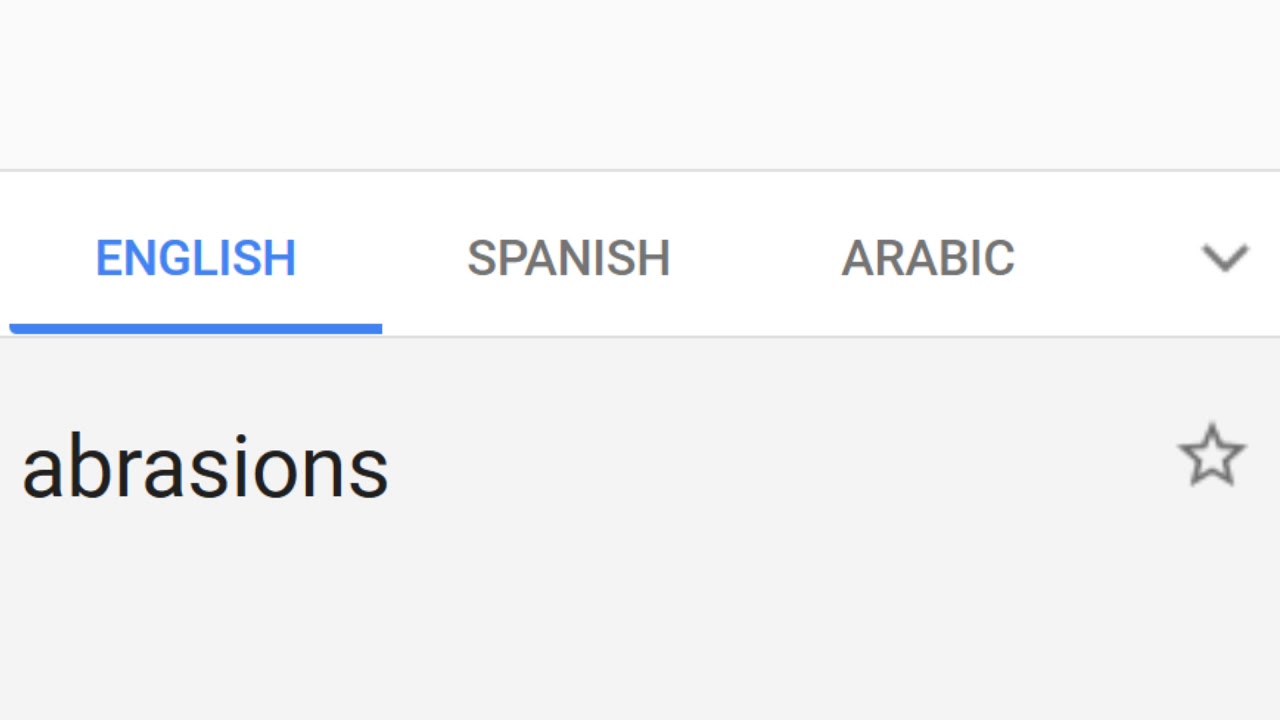This screenshot displays a clean and minimalistic header layout. The header consists of a white stripe with three language options listed on the left side: "ENGLISH" in blue, underlined, and in all caps; "SPANISH" in gray, in all caps; and "ARABIC" in gray, also in all caps. Beside the language options, there is a small down arrow indicating a dropdown menu. Below the header, there is a word in lowercase black font that reads "abrasions," slightly larger in size than the text in the header and without any spaces in between the letters. On the far right side of the same row, there is a star icon with a dark gray outline. The rest of the image is blank, emphasizing the simplicity and focus of the header content.